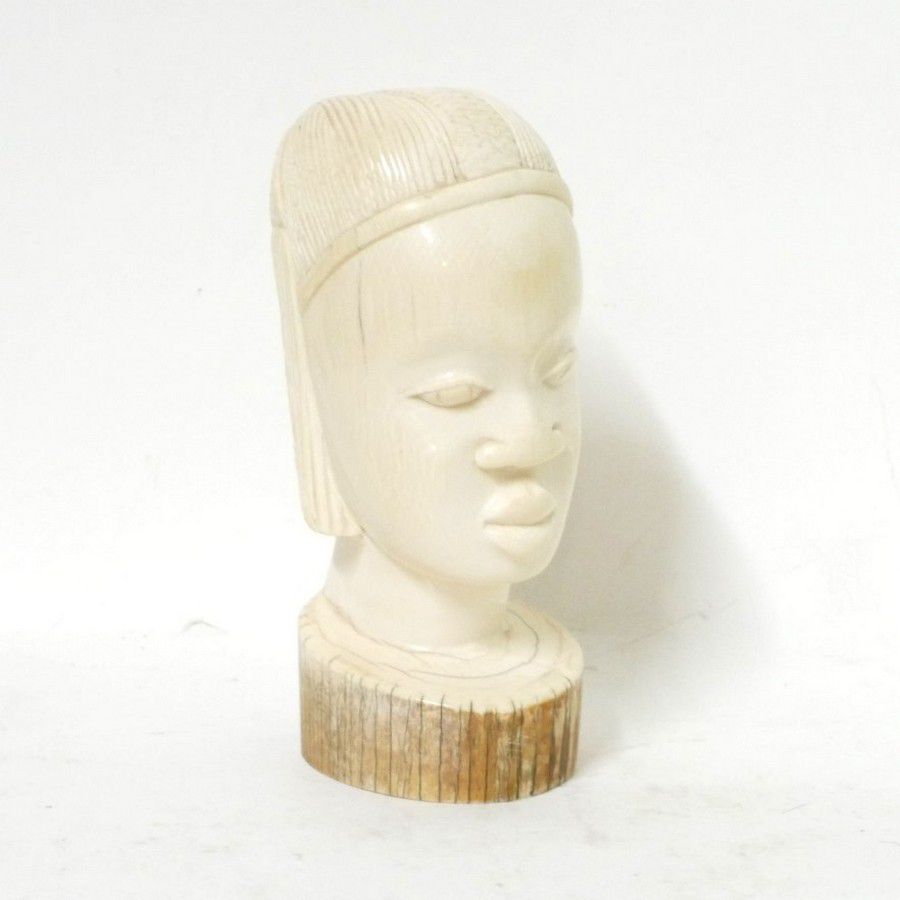The image depicts an intricately carved statue of an African head, likely made from ivory or white wood, giving it a rustic appearance that hints it may have once been a tusk. The head is elongated and oval-shaped, resembling an egg, with a prominent, tall forehead. The facial features include a pair of carved eyes that look to the right, a pronounced nose, and thick lips, indicating it might be a representation of a woman. The statue also features a headpiece, possibly a cap or veil, which adds to the cultural significance. Around the neck, there appears to be a necklace. The head is mounted on a base resembling a cut piece of wood or tree bark, providing a stark, natural contrast to the detailed carving. The entire piece rests against a white background, emphasizing its form and features.